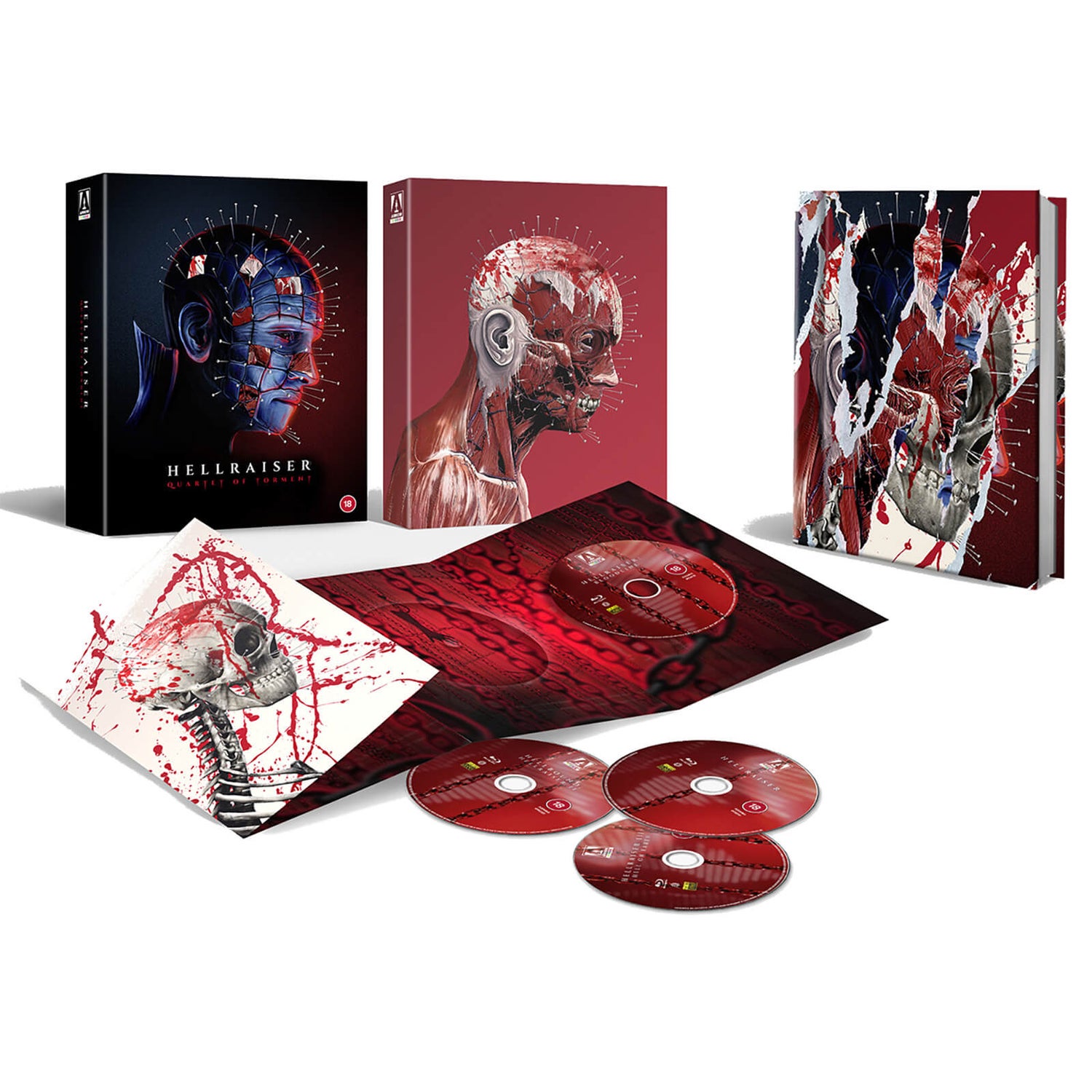This image showcases a deluxe, special edition DVD collection for the movie "Hellraiser.” The collection features a striking morbid design, predominantly using red, black, and white hues with notable blood and pin motifs, invoking the iconic aesthetic of the franchise. At the center of the composition is the main outer box adorned with the classic Hellraiser image, which transforms through varying stages of decomposition to a skeleton on the inner box and accompanying booklet.

At the top of the image, three box designs that resemble books are arranged, each marked with the Hellraiser name. Just below these, there are four red, blood-streaked discs, displayed against a plain white background, contributing to the morbid theme. The middle section showcases an unfolded pamphlet with one distinct red disc on the right and more intricate artwork, including a single skull and streaks of red, emphasizing the skeletal motif further. Additionally, this edition includes a black book, which likely delves into the making of the movie or its artwork, contained in its own sleeve.

Throughout the collection, details such as the blue face with spikes—iconic to Hellraiser lore—are visible, with various iterations of skulls and skeletal imagery depicted in haunting red, white, and black backgrounds. This collection is not only a visual treat for fans but also suggests rich content, possibly including multiple movies and special features. This special edition is a must-have for Hellraiser enthusiasts, given its deluxe presentation and limited availability.